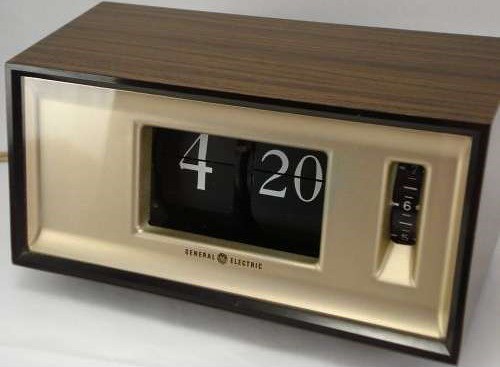The photograph features a rectangular digital clock prominently situated on a white surface. The clock's casing is crafted from dark brown wood, providing a contrast to its cream-colored front face. Centrally located on the clock's face is a black window displaying the time "4:20." Below this window, "General Electric" is written in black text. To the right of the main time display, there is a smaller, thinner black window that houses a dial, which is currently set to the number 6.